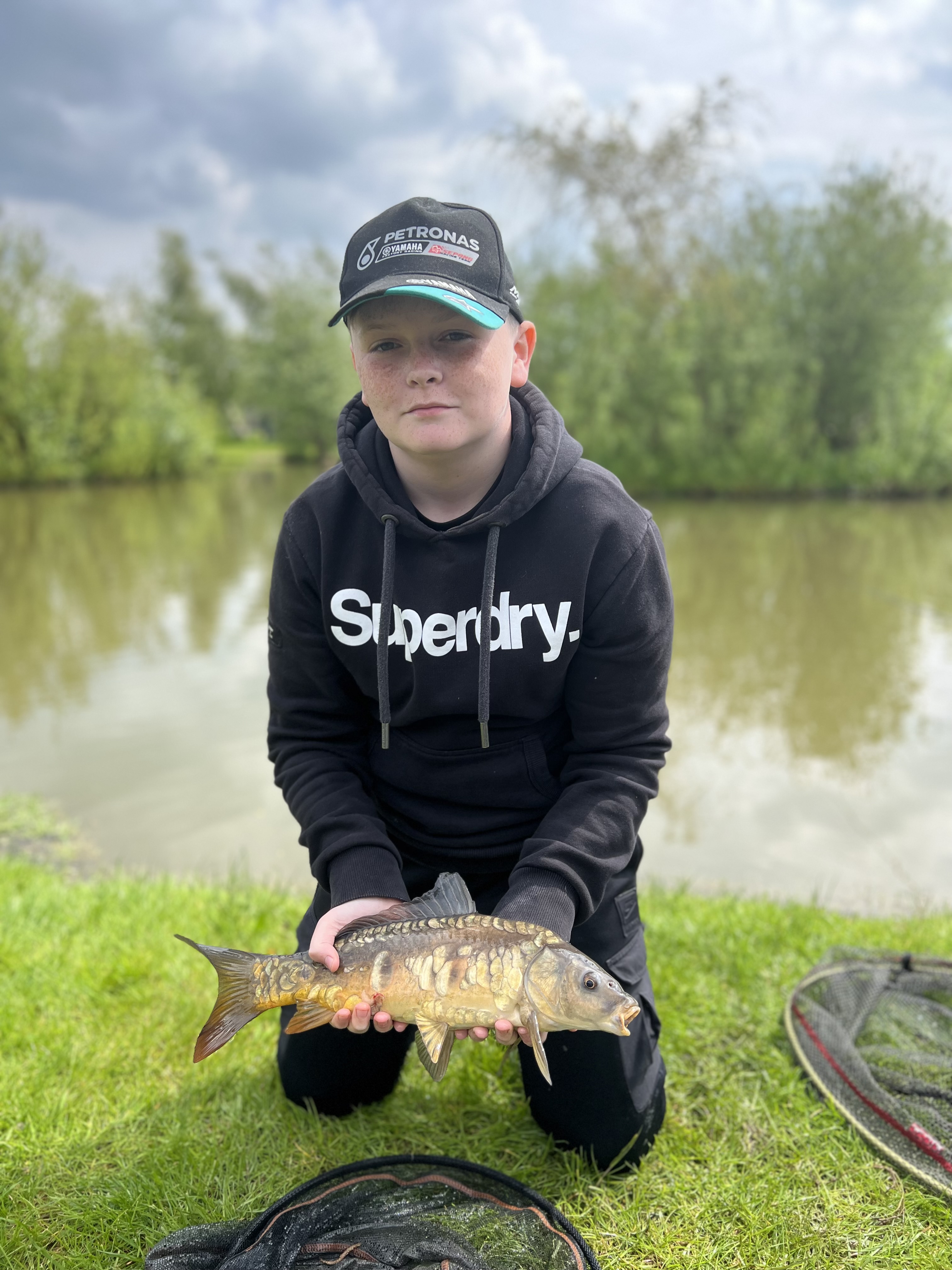In this candid, vertically-oriented photograph, we see a young boy, likely aged between 9 and 11, kneeling on a grassy knoll while proudly holding a fish with both hands. The boy, dressed in black pants and a black "Super Dry." sweatshirt, pairs his outfit with a black hat featuring a turquoise brim. His slight smirk and shiny eyes convey a mix of pride and an attempt to look cool for the camera. The fish, which he holds from a side angle, has a distinct coloration of dark brown with yellow patches. In the foreground, there are nets scattered around, hinting that the fish was recently caught. Behind the boy, a murky pond reflects the surrounding green trees and a sky dotted with rolling clouds, creating a picturesque and natural setting. The composition suggests a spontaneous, casual snapshot, likely taken by a proud parent capturing their child's moment of triumph in nature.